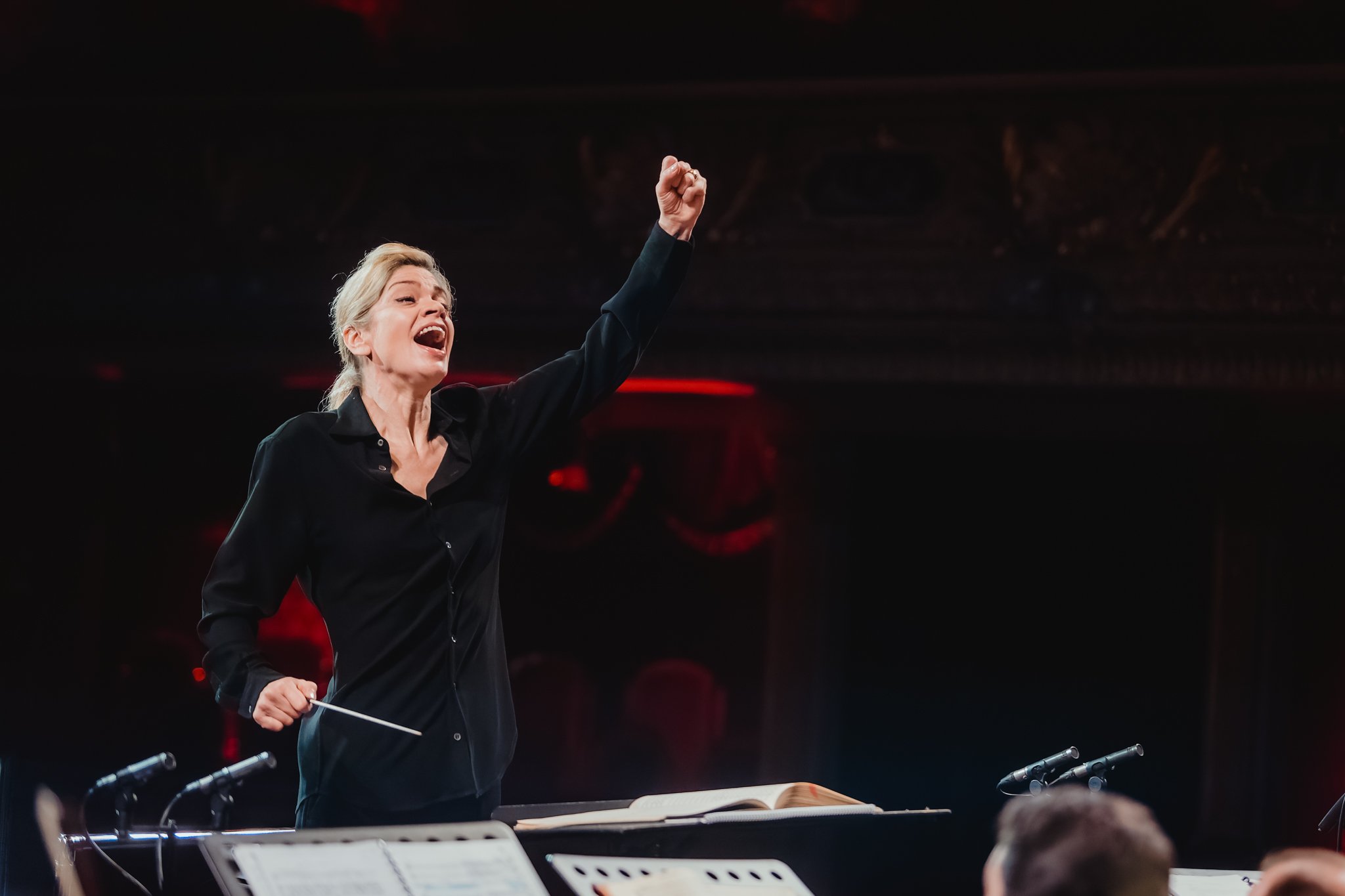In this image, we see a female musical conductor, possibly in her 40s or 50s, energetically directing a choir. She has blonde hair and is wearing an all-black outfit, including a long-sleeved shirt. Her left fist is raised in the air while her right hand holds a conductor's baton. Her mouth is open wide, showing her teeth, as if she is passionately singing or giving instructions to her choir. In front of her, there are several black music stands with white open books placed on them, along with black microphones. The background is predominantly dark, with red lighting that adds a dramatic tone to the scene, and possibly a red chair can be seen. In the bottom right corner of the image, two heads are visible, one with gray hair and one with blonde hair, indicating the presence of choir members. The setting gives a clear sense of being on a stage, with the conductor fully immersed in her role as a maestro.